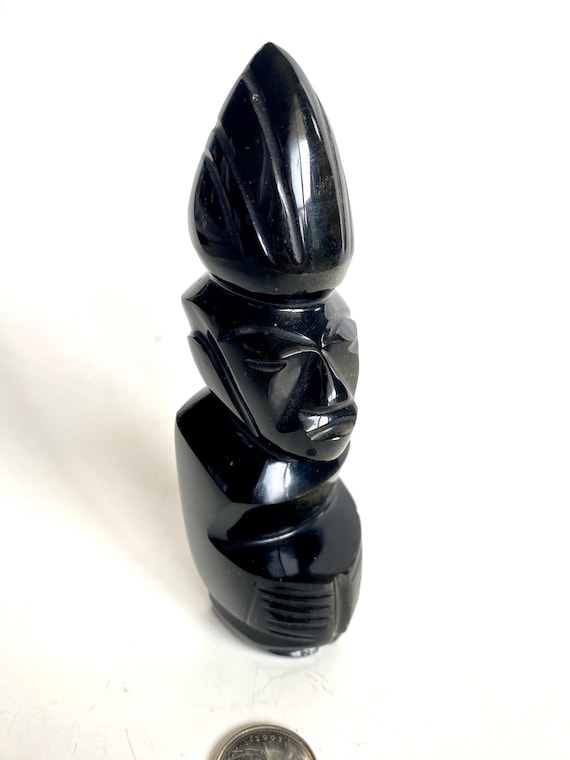The image showcases a detailed black sculpture resembling a chess king piece or a stylized butt plug, resting on a clean, white surface. The sculpture is adorned with the face of a man and features a pointed top, giving it an intricate and artistic appearance. The object is centered in a vertical, rectangular frame and slightly angled to the right. The backdrop is a neutral, off-white color, and the sculpture appears shiny, indicative of materials like resin, stone, or wood. The photograph is likely taken indoors with a focus on highlighting the intricate details and unique design of the piece.